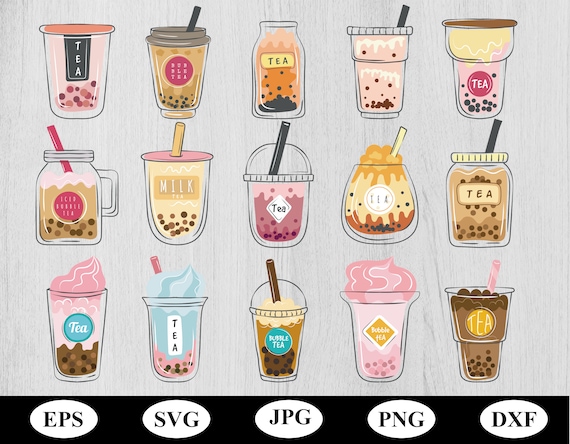The image showcases an assortment of clip art illustrations of various drinks, primarily boba teas and other tea beverages, arranged in three rows and five columns. Each column is categorized under different file format labels displayed at the bottom in a black border with white ovals, specifically EPS, SVG, JPG, PNG, and DXF. The drinks are depicted in a range of colors and flavors, including pink, brown, beige, and orange, and are presented in various cups and glasses, some with lids and some without. Several cups feature whimsical toppings like whipped cream and chocolate drizzles, while others are adorned with straws. Notably, some cups have labels in English and Chinese, indicating different flavors like strawberry, vanilla, chocolate, and mocha, emphasizing the high-quality and diverse nature of these graphic representations.